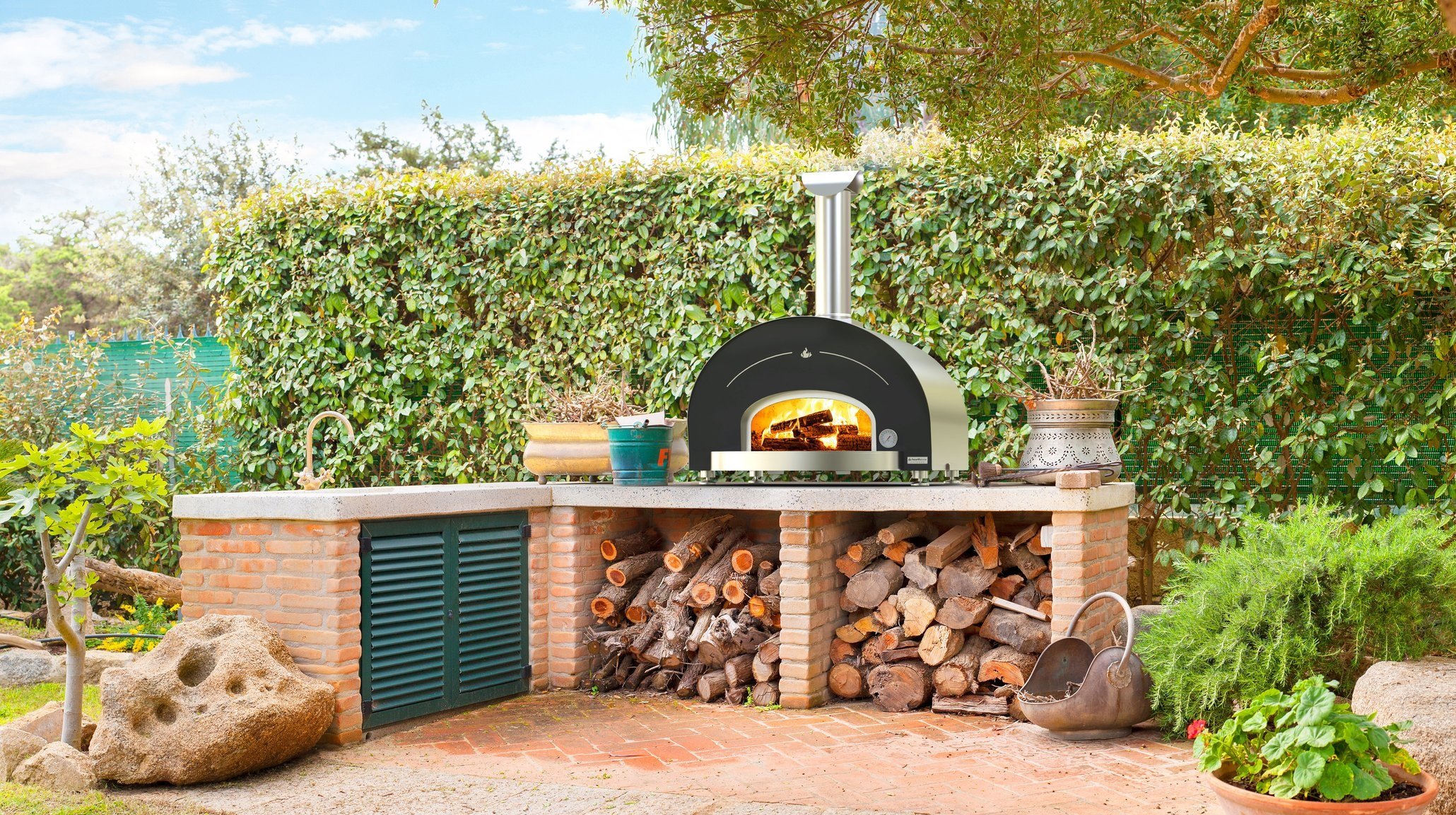In this detailed photograph of a luxurious backyard grilling area, the scene is set on a neatly laid brick patio floor beneath a clear blue sky with scattered white clouds. Central to this outdoor kitchen setup is a sophisticated wood-fire stove, reminiscent of a high-end pizza oven. The stove, housed within an L-shaped brick structure, features a black curved front and a brushed metal dome with a silver chimney extending upwards. Flames and burning logs are visible through the front, emphasizing its functionality.

The left side of the L-shaped counter includes a light beige or grayish countertop with an integrated faucet and sink. Below this section, dark green cabinets with horizontal slats provide storage, while underneath the stove, a neat stack of chopped firewood is visible. Adjacent to the grilling area, a large, hole-riddled sandstone boulder adds a natural touch, surrounded by a selection of small trees and rocks.

In the background, a dense hedge covered in vines, as well as additional shrubs and trees, enhance the garden feel of this sophisticated outdoor space. This entire setup, possibly staged for advertising purposes, exudes an atmosphere of refined outdoor living.